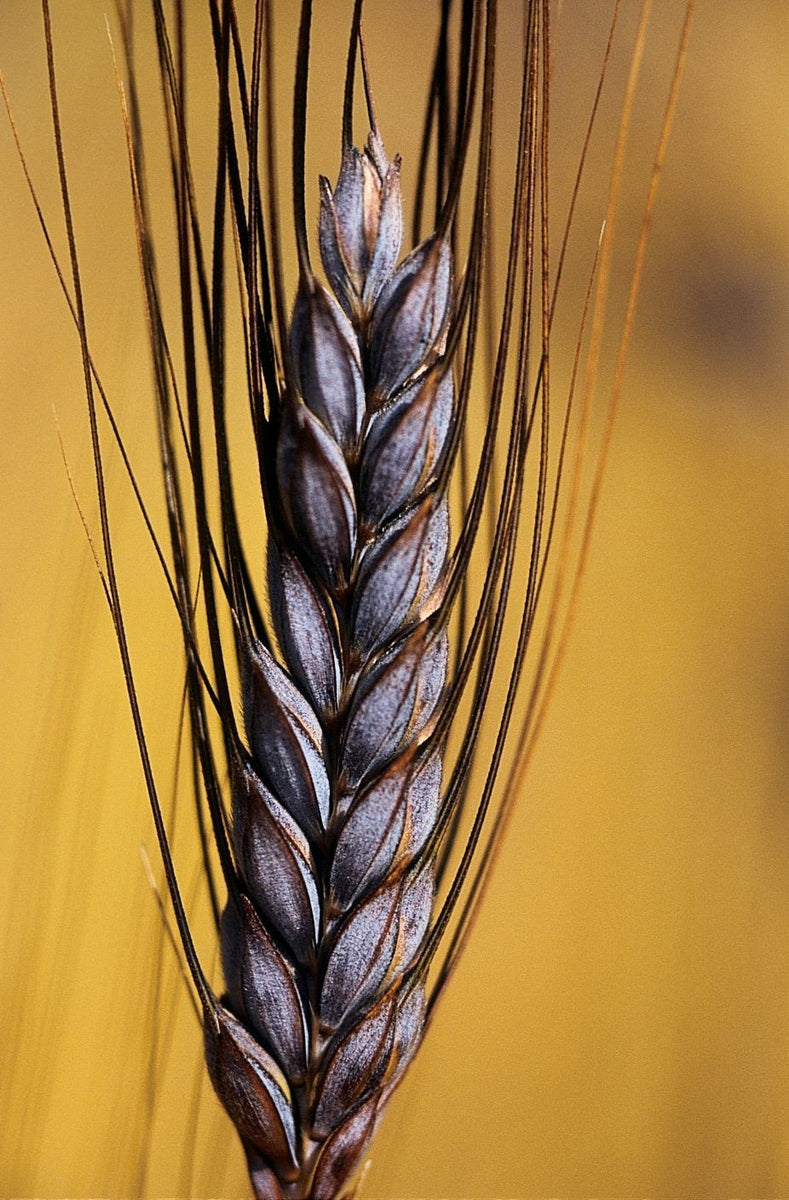This is a vertical, close-up image of what seems to be a single stalk of a unique, possibly computer-animated or edited plant that bears a strong resemblance to a piece of wheat or a reed. The plant is centered in the foreground and extends from the top to the bottom of the image, occupying the entire height. It consists primarily of dark grayish-blue kernels, arranged in a vertical pattern, possibly up to 10 or 15 layers. These kernels are flanked by very thin, dark brown stalks or shoots that give the appearance of needle-like vines. Each seed appears spiky with the topmost kernel beginning to open. The background is a blurry mustard yellow, casting slight shadows of the plant, suggesting it might be either an indoor wall or an outdoor colored scene. However, the blurred nature of the backdrop makes it ambiguous. The vivid description of the plant's structure, the muted background, and the specific detailing of the plant imply a highly focused and intricate portrayal of this fascinating botanical subject.